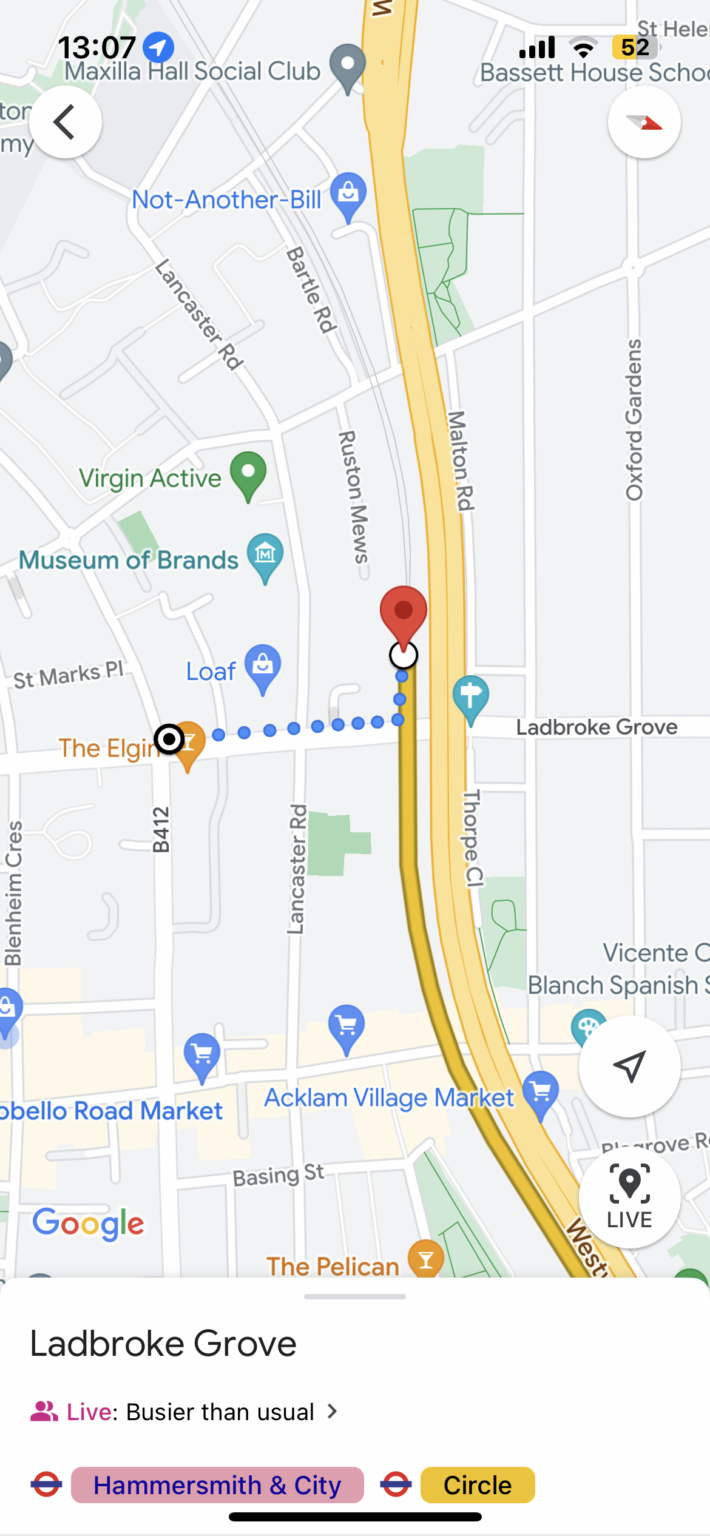A highly detailed screenshot from Google Maps on a mobile phone shows a GPS route. The primary map display features varying shades of gray to denote buildings and landmarks, with darker gray indicating more significant structures. Green patches mark park areas, while blue highlights indicate key locations such as clothing stores and eateries, with one named "Not Another Bill."

Street names are rendered in black. In the upper right-hand corner, the time reads 13:07. The status bar shows a GPS icon on the right side, full Wi-Fi connectivity, and a yellow battery icon indicating 52% remaining power.

The map itself includes a route marked by a line suggesting a subway journey and subsequent walking directions. At the bottom of the screen, “Ladbroke Grove” is displayed in black text, followed by a blue indicator noting "Live," and a black message stating "Busier than usual" with a rightward arrow.

The bottom also features the British Underground logo—a red circle with a white or blue line running through it, symbolizing the subway system. Although the text usually reads "Underground," it is partially obscured. There are labels for the “Hammersmith & City” line as well as the “Circle” line, indicating two potential train routes.